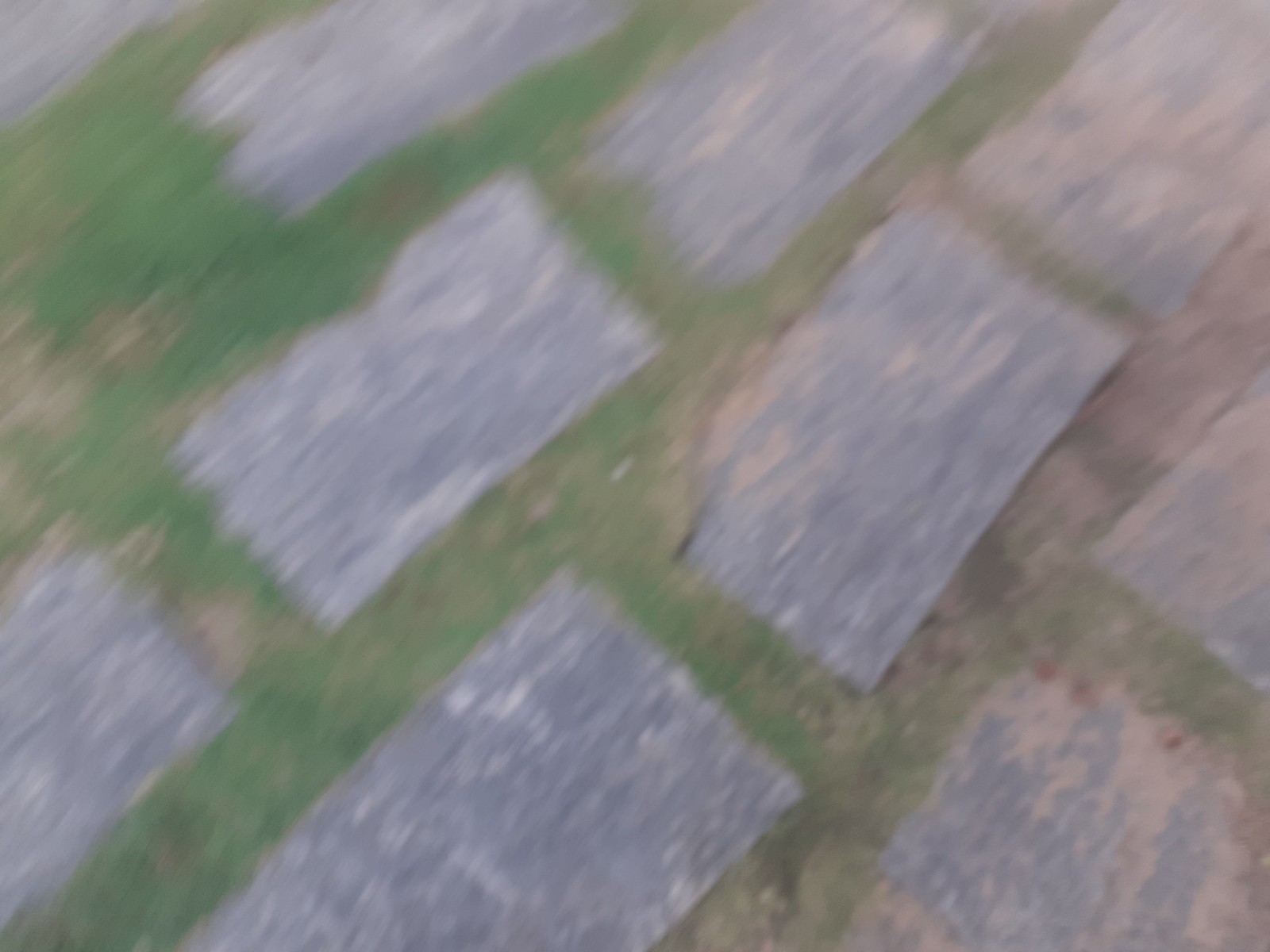The photograph depicts a geometrically arranged path of old, weathered stepping stones or rectangular brick pavers set in a grassy ground area. Although blurry, likely due to motion, the image shows the stones laid in a staggered, zigzag pattern consisting of one stone in the first row, three in the second row, three in the third row, and two in the fourth row. The pavers are spaced approximately an inch apart, surrounded by vibrant green grass interspersed with patchy, brown spots, and bare soil. The stones predominantly exhibit a grayish-white hue, accentuated with sand and dirt, indicating they have been in place for some time. Bright daylight illuminates the scene, suggesting the photo was taken between 1 to 5 p.m. Despite the blurriness, subtle details such as the sand caking on the stones and the grass covering portions of them are visible, contributing to the sense of an aged, well-trodden path.